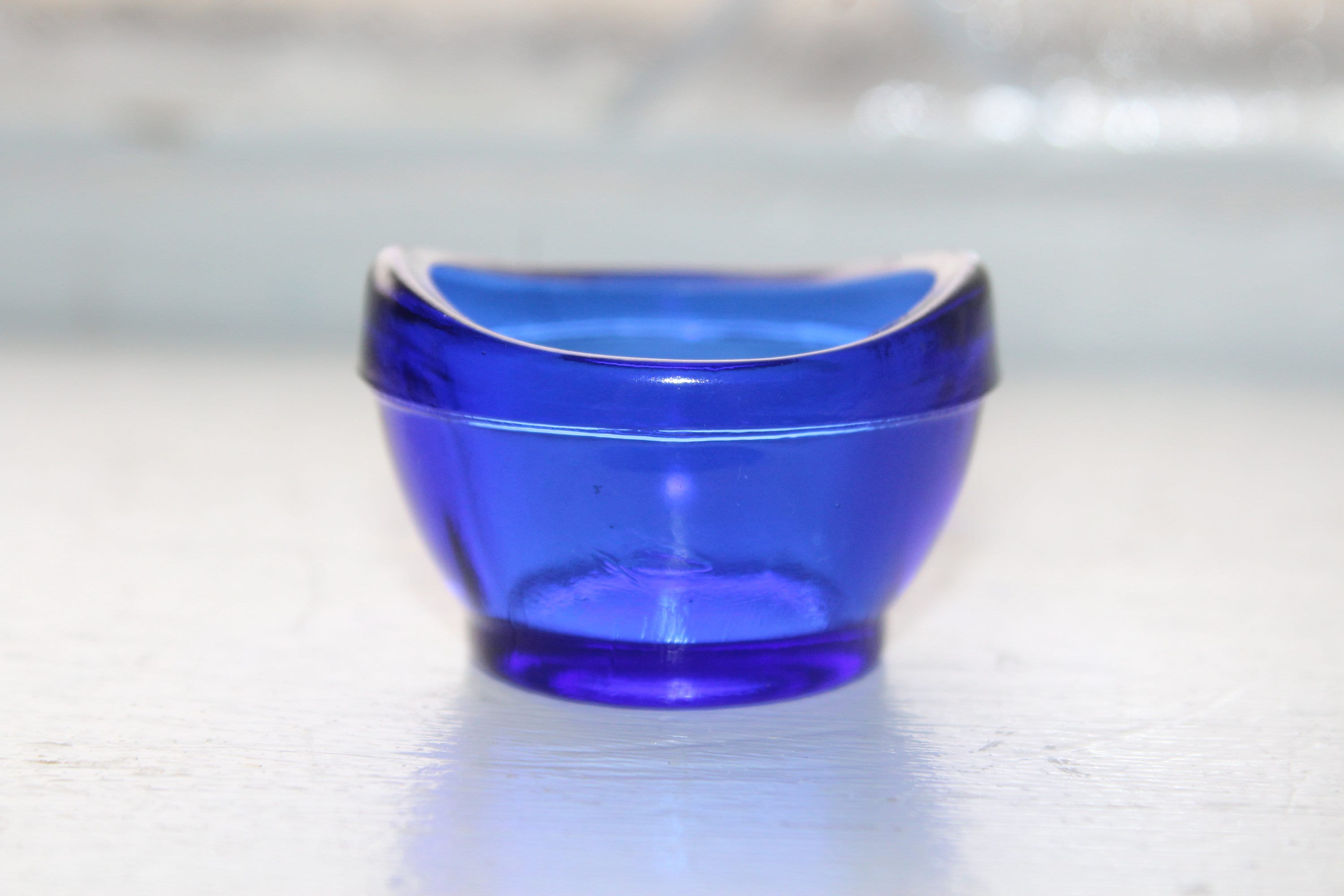The image is an up-close photo of a small, intricate blue container, possibly a jar or bowl, with a complex shape. The container appears to be made of semi-transparent glass, showing various shades of blue; darker at the top and bottom, with a lighter hue through the body. The top of the container features raised sides, higher on the left and right, with a dip in the center, giving a varied profile. It might also resemble a triangular shape and appears to be plastic, but its exact material is unclear. The container is placed on a shiny, white tabletop, which is in focus along with the container. The shadow of the container is visible extending down the image. The background is blurred, displaying a mix of light gray and white tones, suggesting the photo was taken indoors.